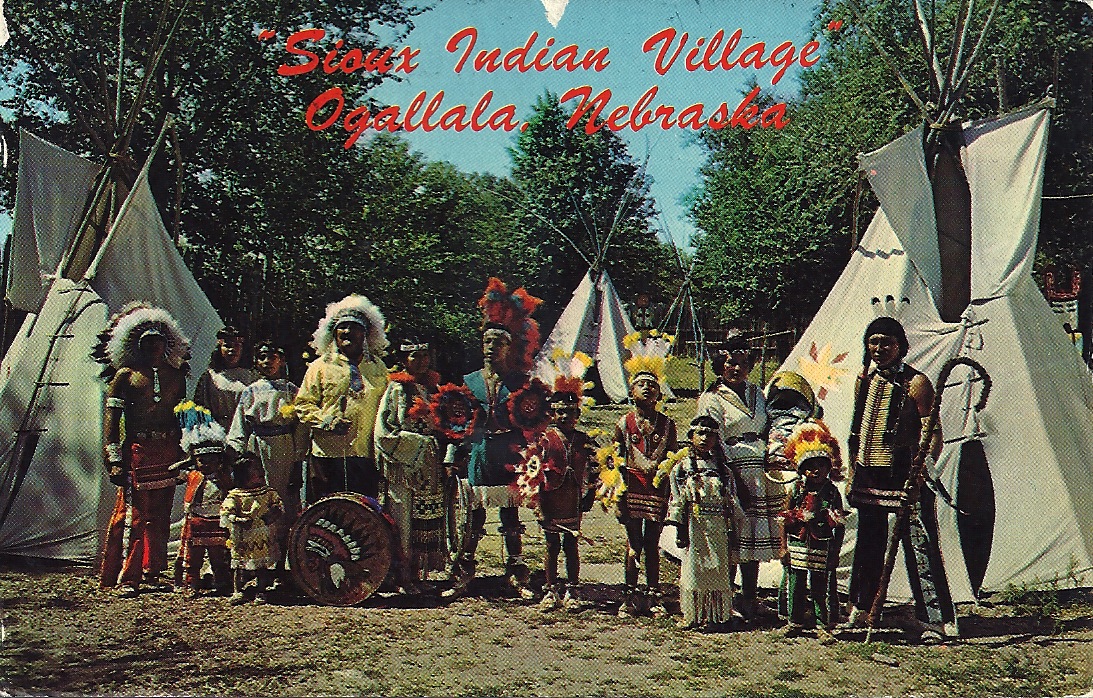This wide rectangular postcard photograph depicts a group of Native Americans standing together in a predominately light brown, dirt, and grassy area with patches of light green grass. The group, consisting of both adults and children—some shirtless and others in traditional clothing—are adorned in bright colors and white feather headdresses, with some headdresses featuring red or yellow accents. Several white teepees, constructed with patterned fabric over arranged sticks, are visible on the left and right sides of the image. The background features tall trees and a bright blue sky visible through the central gap between the trees. Prominently displayed at the top of the image in red, cursive-like font are the words "Sioux Indian Village, Ogalala, Nebraska." In the foreground, there's a large drum bearing the image of a Native American in a headdress with black feathers. Among the group, a young girl wears a yellowish calfskin skirt, and on the far right, a Native American man holds a curved staff in his left hand.